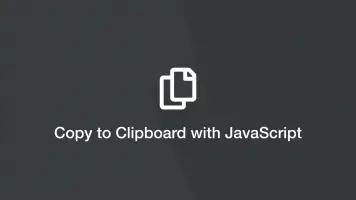A black rectangle measuring approximately 3 inches in height and 4 inches in length dominates the background. In the center, there is an illustration featuring two overlapping pieces of paper, both outlined in white. The top piece of paper is positioned slightly higher, with its upper-right corner bent downwards. The text "Copy to clipboard with JavaScript" is clearly written in white on this top paper. This visual element appears to be an icon related to JavaScript, possibly indicating a functional feature or instruction to copy text to the clipboard. The overall composition suggests that it could be an element from an advertisement or a user interface guidance.